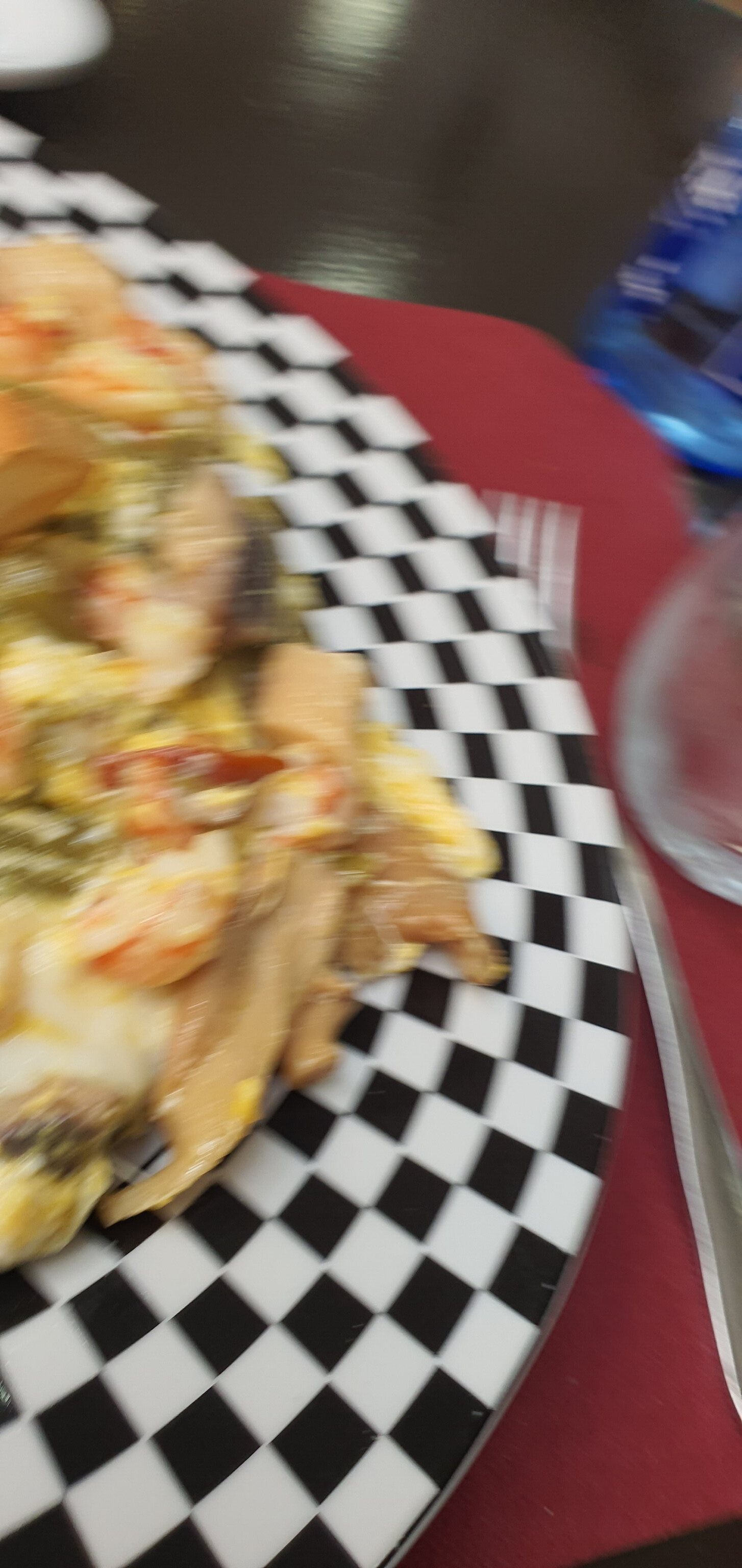In this extremely blurry close-up photograph of a meal, a portion of a large dinner plate rests on a red wine-colored placemat. The plate features a distinctive black-and-white checkerboard border and sits on a possibly black-painted or dark wood table. To the right of the plate, a silver fork peeks out, partially obscured by the plate, alongside a sweating clear glass of cold water. On the far corner of the placemat, part of a blue plastic water bottle is visible. The meal itself appears to be a heaping mound of food, possibly a mix of shredded chicken, baby shrimp, red and green bell peppers, cheese, black beans, and rice, suggesting it could be a burrito or some sort of stir-fry or omelette. The elements are all mixed together, creating a rich and possibly oily and cheesy appearance.